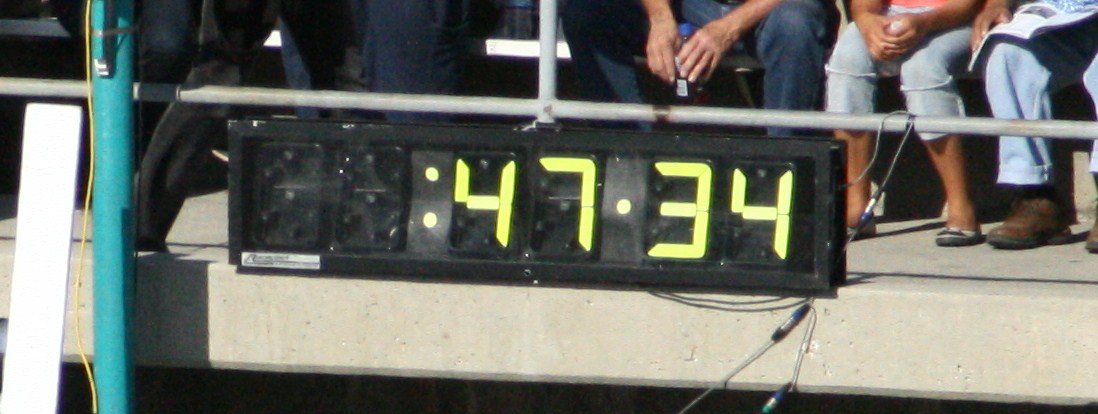This photograph captures a brightly lit, sunny day at a stadium or outdoor event. Central to the image is an electronic timer mounted on a silver metal beam, which displays "47:34" in yellow numbers against a black background, indicative of 47 minutes and 34 seconds. A small white label, likely containing manufacturer information, is visible at the bottom left of the timer but remains illegible. Below the timer and in the foreground are spectators seated casually; though their faces are obscured, their legs and hands resting on their knees are visible. They're surrounded by a metallic railing and various wires connected to the timer, adding an element of electrical setup to the scene. The vivid sunlight flooding the area suggests it's a pleasant and clear day, enhancing the relaxed and casual atmosphere among the viewers.